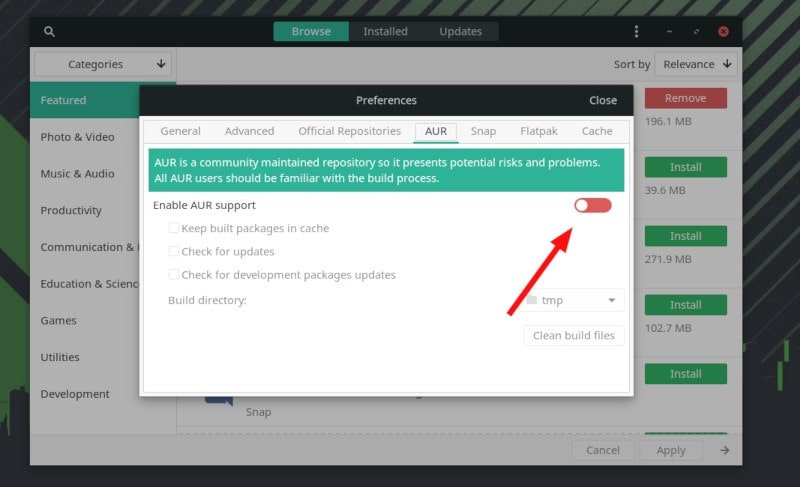The image displays a menu preferences settings window, set against a backdrop featuring alternating light gray and light green lines, with some larger green lines coming in from the left. The pop-up window in the foreground is labeled "Preferences," and it sits atop another window. In the top-right corner of the preferences window is the "Close" button. The bar at the top of this preferences window is black. Directly below this bar is a menu, under which lies a green bar containing important text.

The green bar includes the following information: "AUR is a community-maintained repository, so it presents potential risks and problems. All AUR users should be familiar with the build process." Below this green bar is a red arrow highlighting a toggle switch, which is currently set to the off position, pushed to the left. The toggle, indicated in red with a white button, is meant to enable AUR support when turned on.